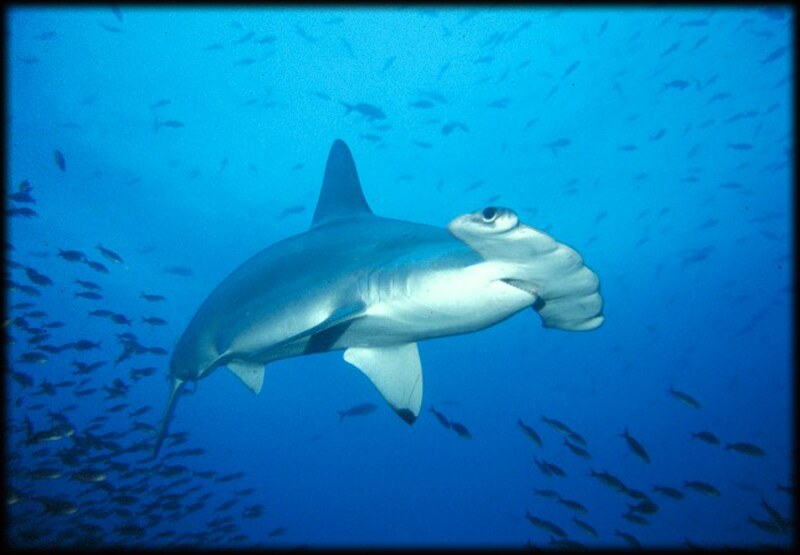The image showcases a hammerhead shark elegantly swimming in the blue ocean, surrounded by an abundance of tiny fish. The shark, with its white underbelly and pearl-like blue and gray body, is oriented towards the right. A significant concentration of fish is visible in the lower-left part of the image, while smaller, less distinct fish populate the upper part, creating a sense of depth. The hammerhead's distinct side eye and mouth are prominently featured, adding more character to the scene. The entire image is framed by a black border, and a notable bright light source illuminates the shark's underbelly, enhancing its detailed textures and colors against the vivid blue water.